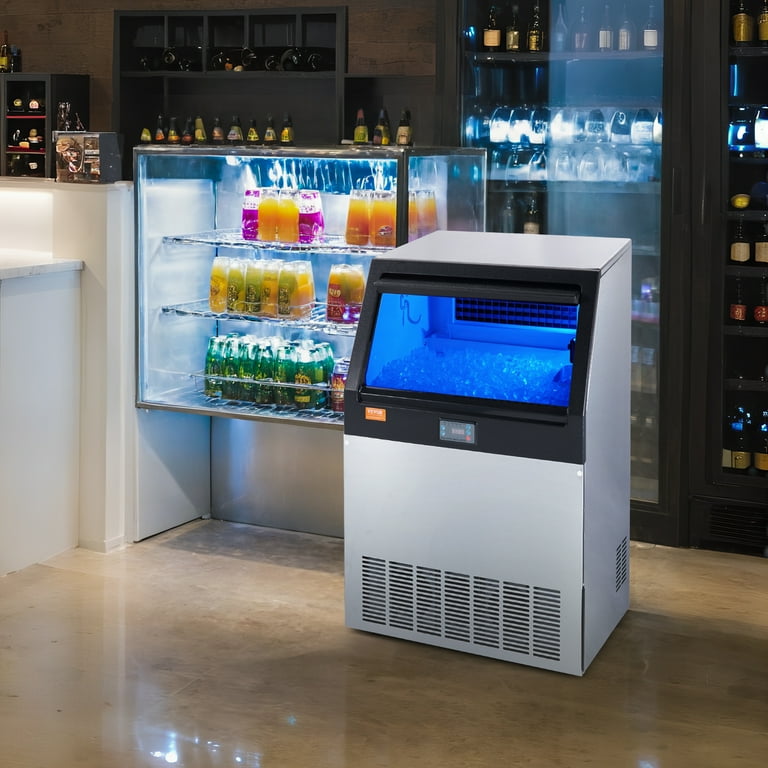In this square photograph taken indoors, the scene is reminiscent of a cozy restaurant bar or coffee shop, likely captured during the evening or nighttime given the dim ambiance. Dominating the center of the image is a refrigerated display case, brightly lit to showcase an array of beverages. This fridge features three distinct rows of drinks: the bottom row houses green glass bottles, the middle row is filled with orange and yellow-hued bottles, and the top shelf is similarly populated with orange-colored drinks, their labels blurred and unreadable. Adjacent to this is an ice maker, visible through an open window that reveals a large container brimming with ice, complete with a handle for scooping. In the background, a glass-fronted shelving unit made of dark wood adds a touch of sophistication, holding various glasses and drinkware, contributing to the overall inviting and warm atmosphere of the establishment.